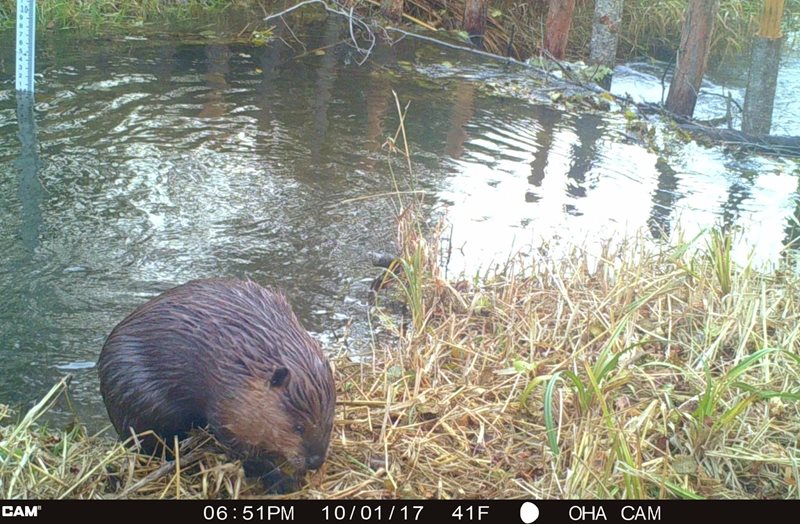This image, captured by a wildlife camera, features a detailed scene along the embankment of a creek or river. A wet beaver, presumably having just emerged from the water, is positioned on the left side of the foreground. The beaver, with its head facing the camera and backside towards the water, is surrounded by a mix of green and tan tall grass, including some mowed down patches. In the background, the water reflects the sky and contains a few ripples, indicating a gently flowing current. There is also a partially constructed dam made of sticks and logs standing upright, with twigs and debris caught in it. Near the top left of the water, a measuring stick is visible. The bottom of the image contains a black rectangular strip displaying the details: "CAM 0651 PM, 10-1-17, 41°F, OHA CAM."